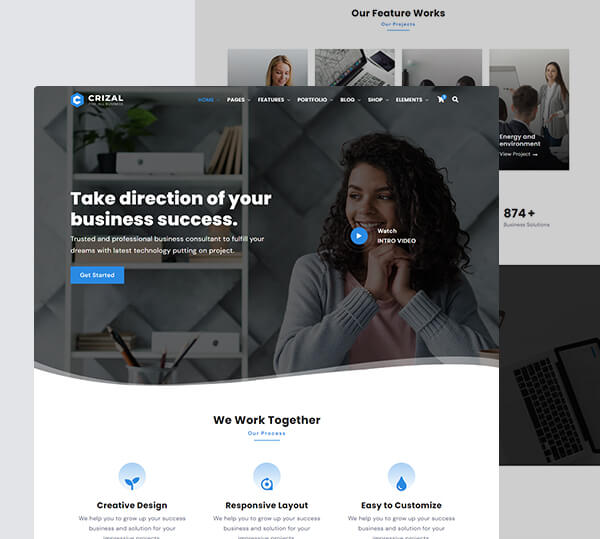A woman is seated with her hands clasped in front of her, her elbows resting on a table in an office setting. The image is part of an intricate collage comprising two superimposed boxes. The top box prominently displays the bold text "Our Future Works" accompanied by two sets of blue lines underneath, labeled "Our Project," though the text gets partially cut off. This box features four different images: one shows a blind woman with medium-length hair looking down at a monitor and keyboard with a phone beside it. Another glimpse reveals the heads of individuals, possibly engaged in a meeting. A third image portrays a woman in a long dress with long sleeves, standing by a white easel, appearing to lead a business presentation. The text "874+" can be seen near this section.

The second box, fully visible, features the heading "CRIZAL" with a blue "C" badge logo on the left. The navigation menu includes options such as Home, Pages, Features, Portfolio, Blogs, Shop, and Elements, with drop-down menus, and the Home option highlighted in blue, indicating the current selection. To the right of the menu, there are icons for a shopping cart and search function. Beneath this, in a prominent font, reads "Take Direction of Your Business Success," followed by the smaller text, "Trust a professional business consultant to fulfill your dreams and latest technology putting on a project." Below this message, there are "Get Started" and "Watch Intro Video" buttons. The lower section includes the phrase, "We work together," followed by details on creative design, responsive layout, and easy customization.